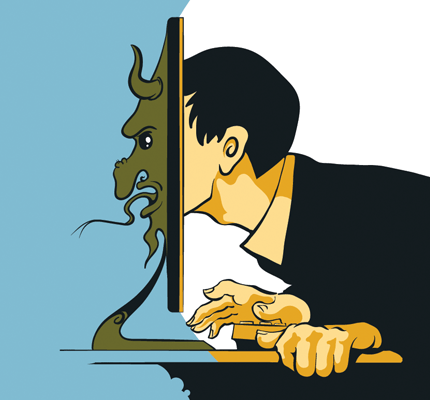This detailed digital drawing showcases a man with black hair and a yellow-collared black jacket, positioned on the right side, where he appears to be pressing his face through a computer monitor. His hands grip the edge of a desk with a keyboard, which is linked to a monitor displaying a side view with a base arm extending backward. The right half of the image features a white background and depicts the man's normal backside, including his neck and hands.

Contrastingly, the left side of the image morphs into a surreal, light blue background where his face emerges as a grotesque green devil. This devilish face includes details such as brownish-green skin, sinister horns, a long, wart-covered elongated nose, a forked serpent-like tongue, and a small goatee. The scene conveys a metaphorical transformation as the man's normal visage transitions dramatically into the devilish figure, hinting at an artistic exploration of duality or inner demons through the merging of mundane and fantastical elements. Various colors like black, yellow, green, light blue, white, and brown enhance the striking visual contrast in the image.